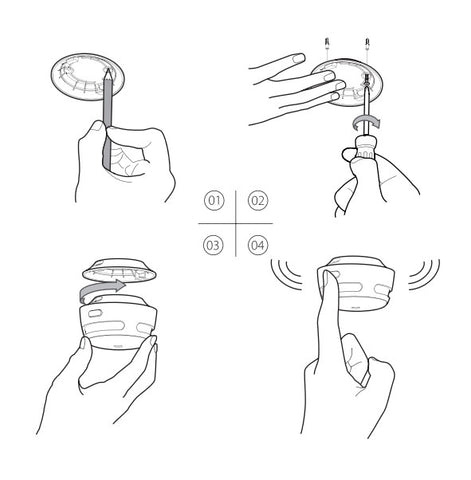The image is a detailed instructional drawing illustrating a step-by-step guide on how to install a fire alarm or sensor under a countertop. In Step 1, depicted in the top left corner, a hand is shown holding a pencil, marking the placement spots for the screws by holding the bracket against the surface. In Step 2, shown in the top right, a hand is using a screwdriver to insert screws into the marked spots, securing the bracket in place, with arrows indicating the clockwise direction for tightening. Step 3, in the bottom left, features a hand positioning the main unit of the device into the already installed bracket and turning it counterclockwise to lock it into place. Finally, Step 4, in the bottom right, shows a finger pressing the power button on the device, indicated by sound waves emanating from both sides, suggesting that the device is now activated and operational.